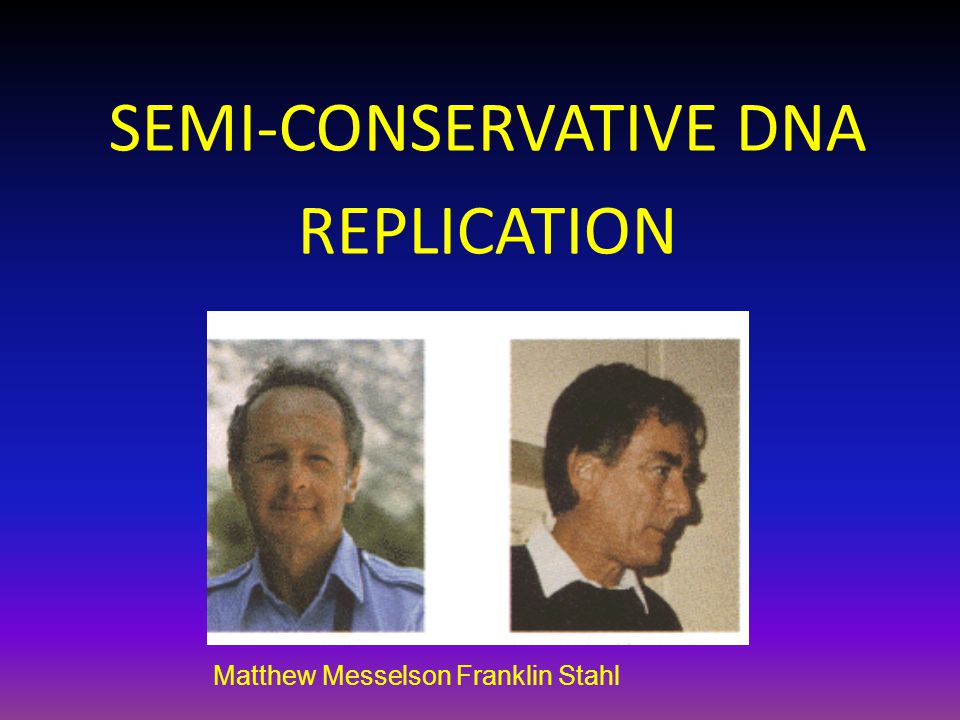The image is a PowerPoint slide featuring the title "SEMI-CONSERVATIVE DNA REPLICATION" in large, all-cap yellow lettering at the top. Below the title, there are two juxtaposed, old grainy photographs of two white men with white borders on the top and right edges. The man on the left is looking directly at the camera, while the man on the right is gazing to the right in a profile shot. Both are dressed in button-down, collared shirts. Beneath their photographs, their names are clearly written: "Matthew Messelson" and "Franklin Stahl." The background of the slide transitions from a dark blue at the top, gradually fading into a lighter blue, and then blending into a purplish-pink hue at the bottom.